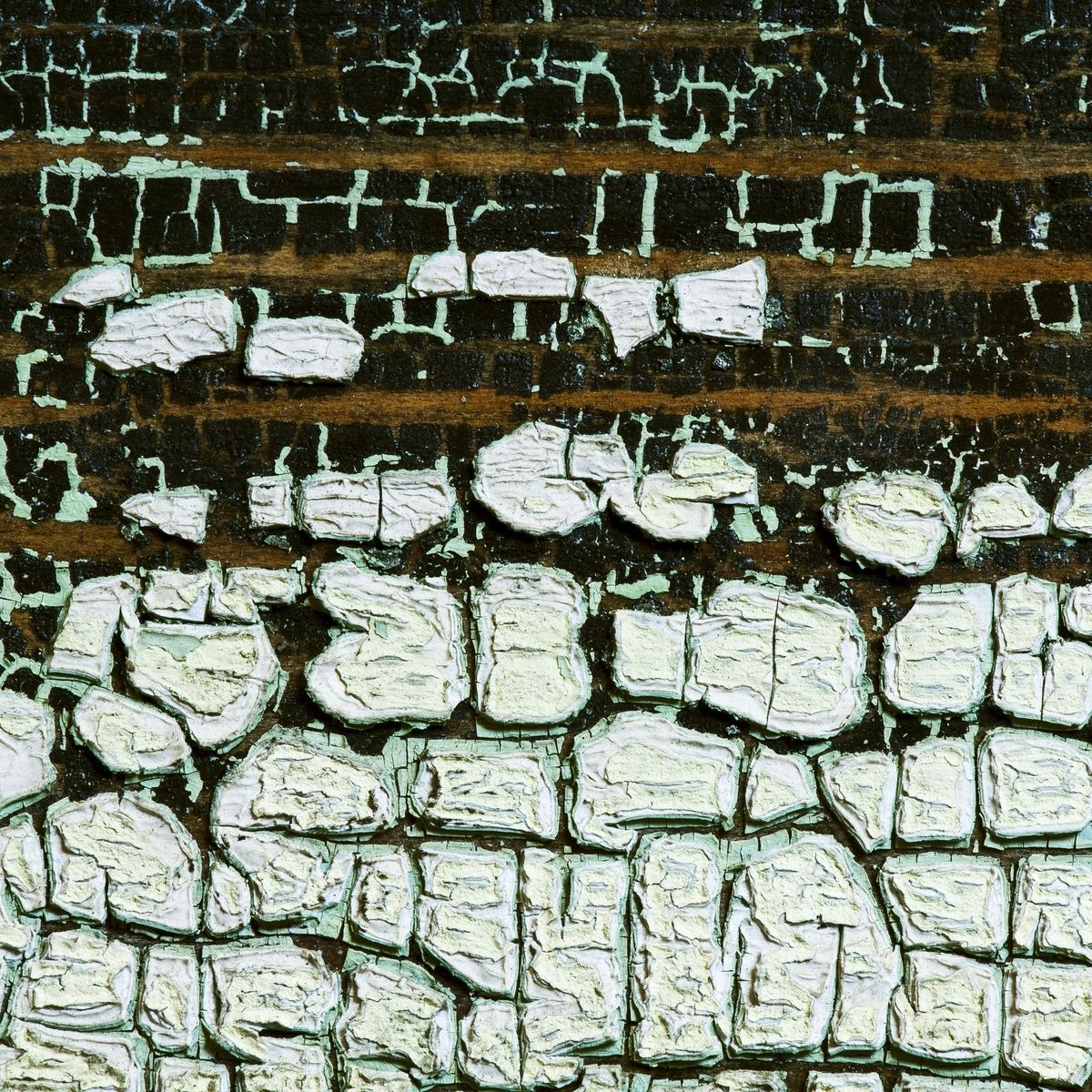This image showcases an abstract artwork characterized by a vertically rectangular canvas with no definitive background. The composition predominantly features cracked and weathered areas resembling old paint on a wall. At the top portion of the image, there are fragments of black paint interspersed with a few gold lines, which run horizontally across the canvas. Moving downward, the artwork is intersected by horizontal brown and light mint green lines, adding rich contrast and a sense of structure. These horizontal lines taper off as they approach the lower portion of the canvas, giving way to larger, pronounced white shapes that have a crumpled, 3D appearance. These sections of white resemble crumpled paper, mingling abstractly within the piece. Additionally, splatters of black are dispersed throughout the image, contributing to its intricate, textured aesthetic. This combination of elements creates a visually engaging and abstract representation that evokes a sense of aged, weathered surfaces and layered complexity.